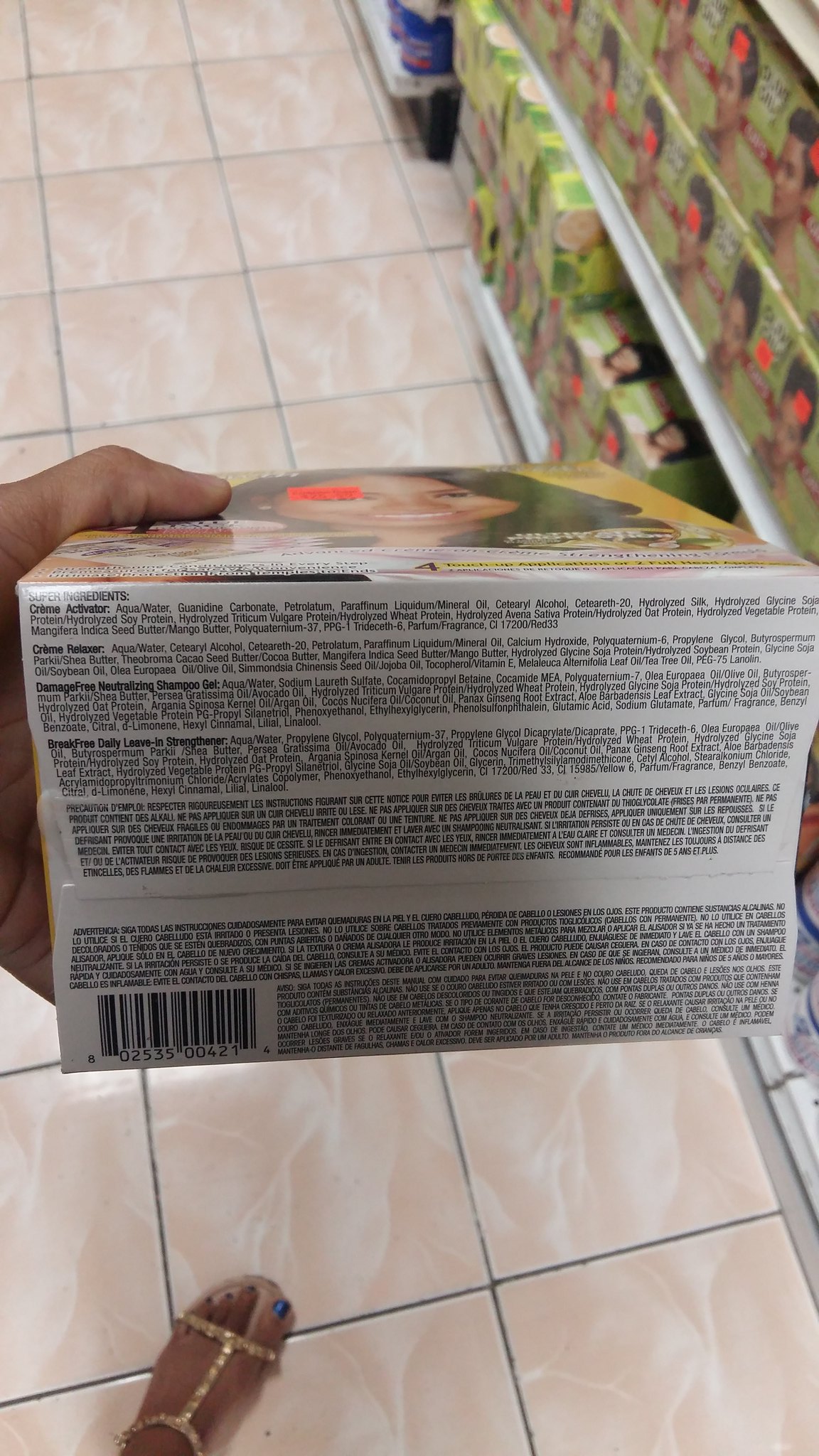A woman with darker skin stands in a retail store, inspecting a box of hair dye from a display shelf filled with various hair color options. She holds the box in her left hand, revealing the product information on the bottom side. The front of the box features a smiling woman with long black hair, and an orange price sticker that matches the stickers on all the other boxes on the shelves. The woman in the store is partially visible, with her right foot in view. She wears a delicate and glittery gold sequin sandal, which has a strip over the toes, another strip up to the ankle, and finally an ankle strap. Her toenails are painted in a bright blue tonal polish. The store's floor is tiled in a pink and white pattern with gray grout between the tiles, adding to the vibrant and colorful atmosphere of the scene.